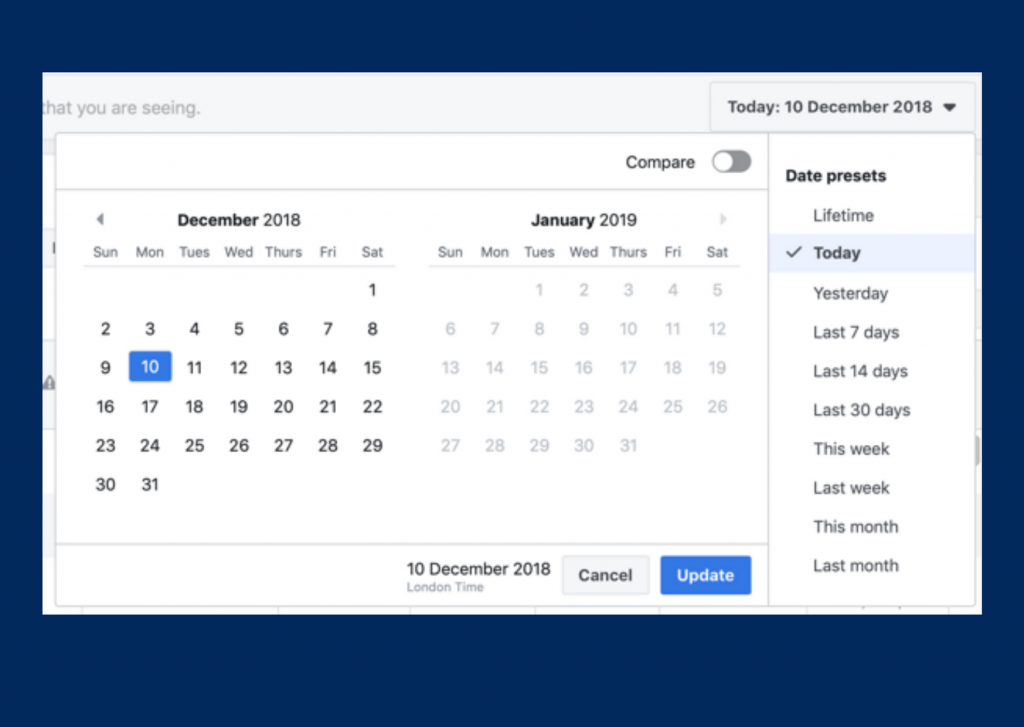The image features a user interface with a dark navy blue background. At the top, a light gray header displays partially cut-off text that reads, "What you are seeing." To the right, there is a rectangular section with a light gray background and a darker gray border. This section contains bold gray text stating, "Today: 10 December, 2018," followed by a filled-in gray arrowhead pointing downwards, suggesting that it is an expandable dropdown menu. 

When expanded, the dropdown menu reveals options on a white background under the title "Date Presets" in bold lettering. The options listed in gray text include "Lifetime," "Today," "Yesterday," "Last 7 Days," "Last 14 Days," "Last 30 Days," "This Week," "Last Week," "This Month," and "Last Month." The "Today" option is selected, indicated by bolded text, a check mark to the left, and a light blue highlight.

On the left side of the interface, the header with a white background contains the word "Compare" in black bold lettering, accompanied by a toggle switch on the right, which is currently off. Below this header is a thin black line divider.

Furthermore, there are two adjacent calendars. The left calendar is for December 2018, with "December" in bold black text and "2018" in non-bold text. The right calendar is for January 2019, with "January" bolded and "2019" not. All dates in the January calendar appear in light gray, indicating they are disabled. The 10th of December is highlighted by a blue square, signifying that it is the selected date.